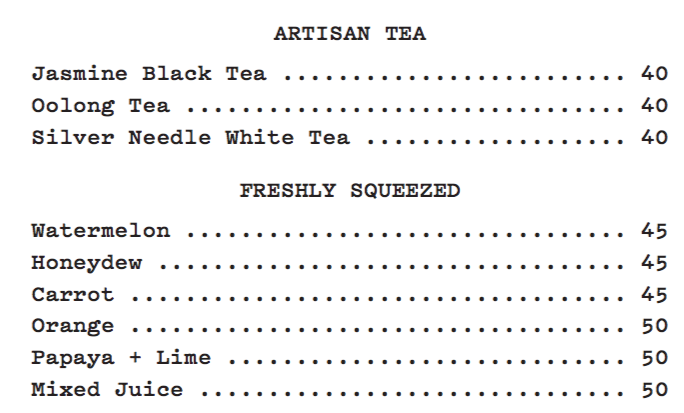The image depicts a simple, white-background menu divided into two sections. The first section, centered at the top, is labeled "Artisan Tea" in black typewriter-style text. It lists three tea options: Jasmine Black Tea, Oolong Tea, and Silver Needle White Tea, each priced at $40. Below, the section titled "Freshly Squeezed" features six juice options: Watermelon, Honeydew, and Carrot, each priced at $45, followed by Orange, Papaya and Lime, and Mixed Juice, each priced at $50. The clean, minimalist design presents the drink choices and their prices in a straightforward manner, with dots possibly used as spacing between the item names and their prices.